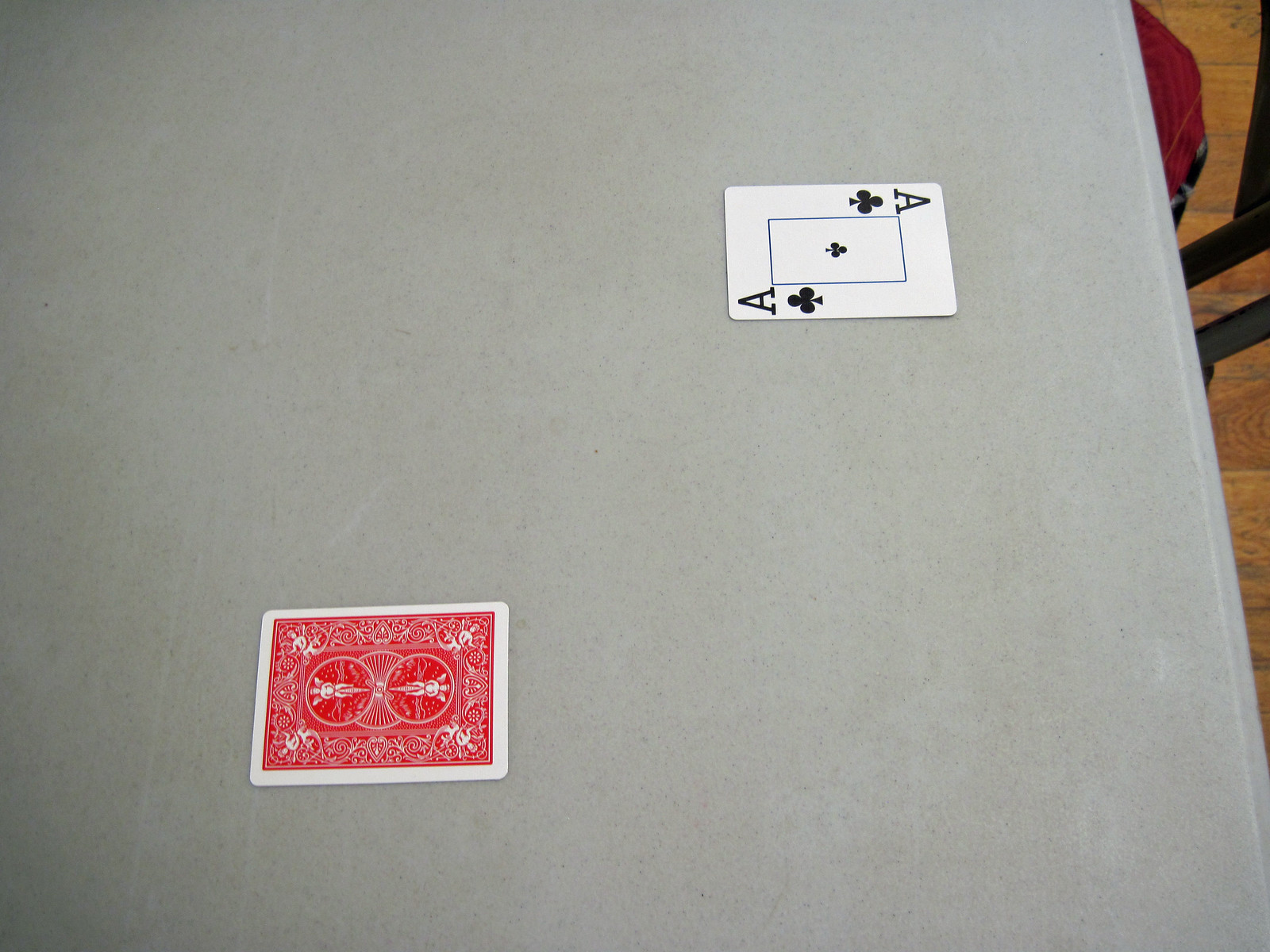The image depicts a simple scene of a white plastic table. On the far right edge of the table, there's a vague glimpse of what could be the edge of a chair partially visible beneath the table. The table holds only two playing cards: in the top right corner, the Ace of Clubs is face-up, displaying its distinctive three-leaf clover symbol in the center. In the bottom left corner, a single card lies face-down, revealing only the classic red back design of a standard deck of cards. The table is otherwise empty, and there are no people present in the photo. The setup suggests the early stages of a card game, possibly blackjack, with the players awaiting the dealer to deal the next card. The overall composition is minimalistic, focused solely on the potential beginning of a game.